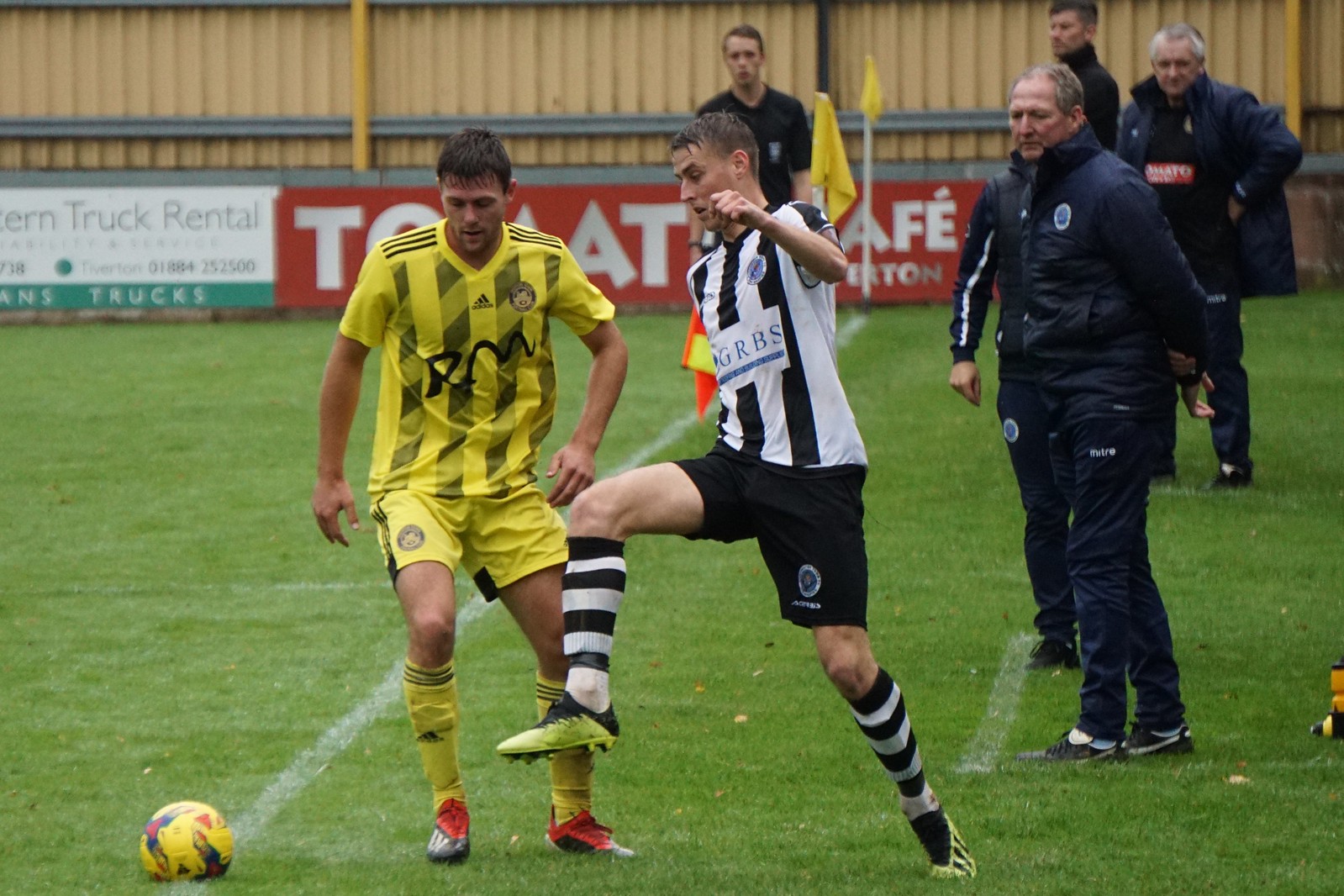In the soccer field image, two players from opposing teams are in the midst of a match. The first player is clad in a yellow uniform featuring a top with light black stripes and matching yellow socks. The second player dons a white jersey adorned with black stripes, black shorts, and black and white horizontally striped socks. A unique yellow ball, possibly not a standard soccer ball, is prominently visible on the field, marked with a logo. Surrounding the partaking players are four men in black attire, likely officials overseeing the game. The backdrop features a tan wall with a support post and a yellow flag positioned on one of the field lines. Additionally, the wall is adorned with two or three financial advertisements, including a truck rental ad in white and green, and another partially visible, possibly for a café, showing a red and white logo with the letters T-O-M-A-T and an accent over an E. The overall scene is characterized by predominant black, white, yellow, and green colors.